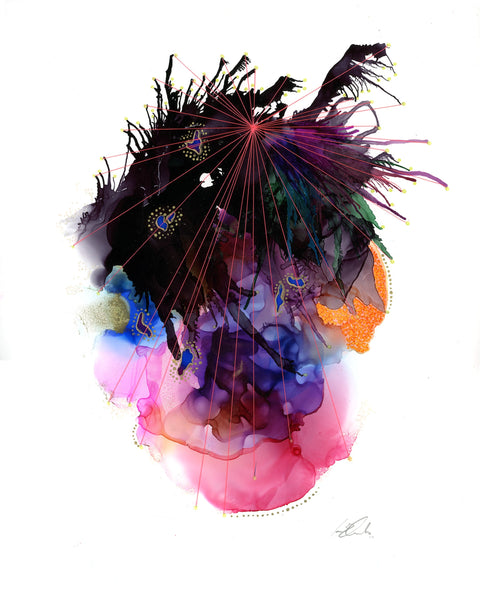On a white background with watercolor gray stripes on the left and right sides, this modern abstract art piece features a central composition full of texture and color. At the bottom, a half-circle of small gray dots serves as the foundation. Above it, there is a cloud of pink that expands into a busy display of purples and blues, resembling crumpled flower petals. To the right side, a vivid bright orange section stands out, while to the left, blues and greens intermix. The top portion of the artwork transforms into dark scraggly branches with moss hanging toward the right. Dominating the topmost center, a large black shape is punctuated by a red light emitting laser-like beams in all directions. Scattered throughout the image are elements that resemble plant parts, including a starburst in purple at the top with string-like extensions, blue blossoms, and an orange leaf. An illegible signature at the bottom hints at the artist's presence. The piece is a visually stimulating blend of shapes and colors, embodying the essence of abstract art.